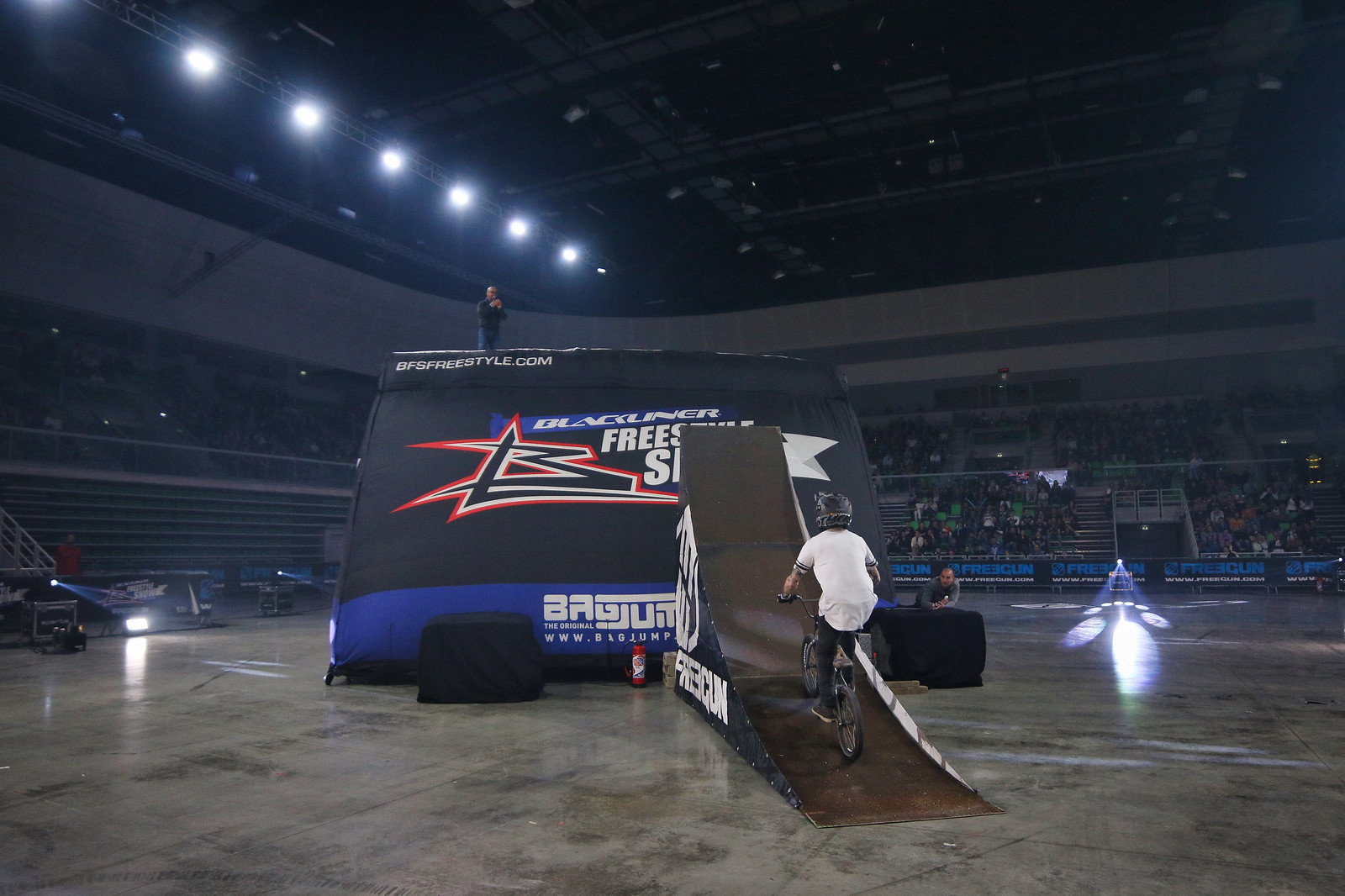The photograph captures a thrilling extreme bicycling event inside a large indoor stadium, typically used for basketball games but now featuring a polished dark gray concrete floor. At the very center of the arena stands an imposing black inflatable obstacle, estimated to be around 20 to 30 feet tall, emblazoned with a prominent red and black logo featuring the letter 'B' and partially obscured text "Black Liner Freestyle." On top of this massive structure, a man holding a microphone stands, possibly a referee or presenter, while another man is positioned at the base. A BMX cyclist, clad in a white t-shirt, black helmet, and black pants, is captured mid-action, riding up a steep, dark brown ramp, clearly preparing for an impressive jump. The cyclist is well-lit by spotlights, underscoring the high-stakes nature of the stunt. In the backdrop, the stadium bleachers are dimly lit, revealing a sizable but shadowy audience eagerly watching the event unfold. The upper rafters of the stadium can also be seen, adding to the grandeur of the venue.